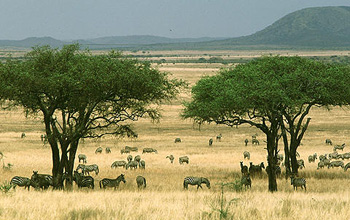The photograph is a low-resolution, pixelated image capturing the vast expanse of an African savannah under a light blue, cloudless sky. In the foreground, there are three thin brown-trunked trees with thick green canopies, providing necessary shade to a large herd of zebras grazing beneath. The flat, largely barren landscape stretches far into the distance, covered in tall yellow-brown grass with only a few sparse trees scattered across the horizon. In the far distance, the horizon is marked by multiple large hills lush with green vegetation. The zebras, distinguishable by their black and white striped patterns, are dispersed across the scene, with some congregated under the trees and others scattered throughout the area, grazing and moving about. The overall bright daylight highlights the dry and arid characteristics of this quintessential savannah landscape.